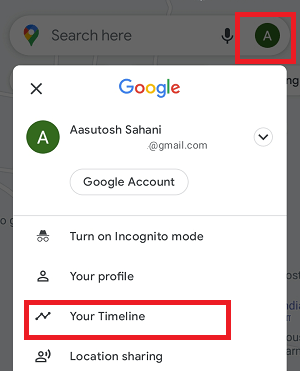The image features a dark gray background with a prominently outlined red square in the center. Inside the red square, there's a capital letter 'A' in white, which is encircled by a green circle. To the left of this square is a microphone symbol, accompanied by a search bar prompt that says "Search here."

Below these elements is a long white rectangle, centered with the word "Google" written in its characteristic multicolored logo: a blue 'G', a red 'o', a yellow 'o', a blue 'g', a green 'l', and a red lowercase 'e'. Within the design of this logo, there is a green circle encompassing a white, capitalized letter 'A'.

To the right of this logo are the letters "A-A-S-U-T-O-S-H" followed by "S-A-H-A-N-I," and underneath this text, in a smaller font, is "at gmail.com." Below this is a large circle containing the words "Google account."

Beneath the circle, a line separates the text "Turn on incognito mode" from the remaining options below. The next segments of text sequentially read: "Your profile," "Your timeline" (outlined in red), and "Location sharing."